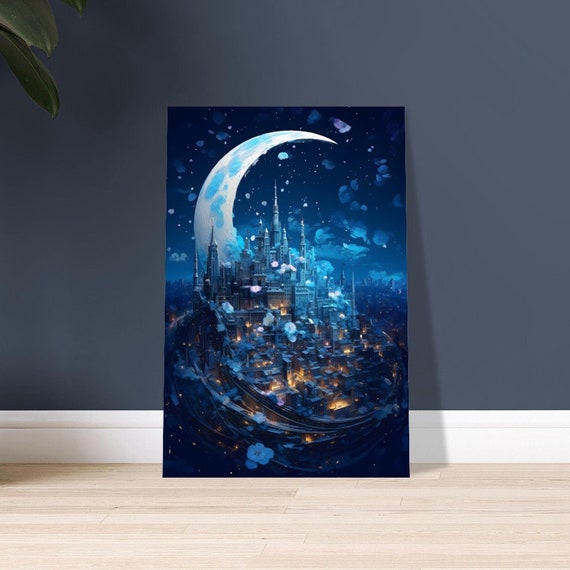The photograph depicts an enchanting, vertically oriented painting of a fantastical cityscape, which leans against a grayish-blue wall adorned with white molding along the bottom. The flooring is light brown wood, creating a soft, inviting contrast to the darker wall color. In the upper left corner of the photograph, a portion of dark green leaves, possibly from a plant, intrudes into the frame.

The mesmerizing artwork features a dreamlike, sky-bound city illuminated with warm, orange lights, suggestive of nighttime. Below this ethereal city lies a grounded skyline, providing a striking dichotomy. Floating above and throughout the surreal city are delicate, flower petal-like forms that enhance its fantastical nature. Dominating the background, a large, intricate crescent moon, tinged with light blue hues for added depth, arcs majestically across the scene. The sky transitions smoothly from light blue to dark blue, finally merging into black, encapsulating the image in a cosmic aura. The painting, rich in textures and dramatic lighting, conjures an otherworldly sense of magic and mystery, reminiscent of a whimsical fantasy realm.